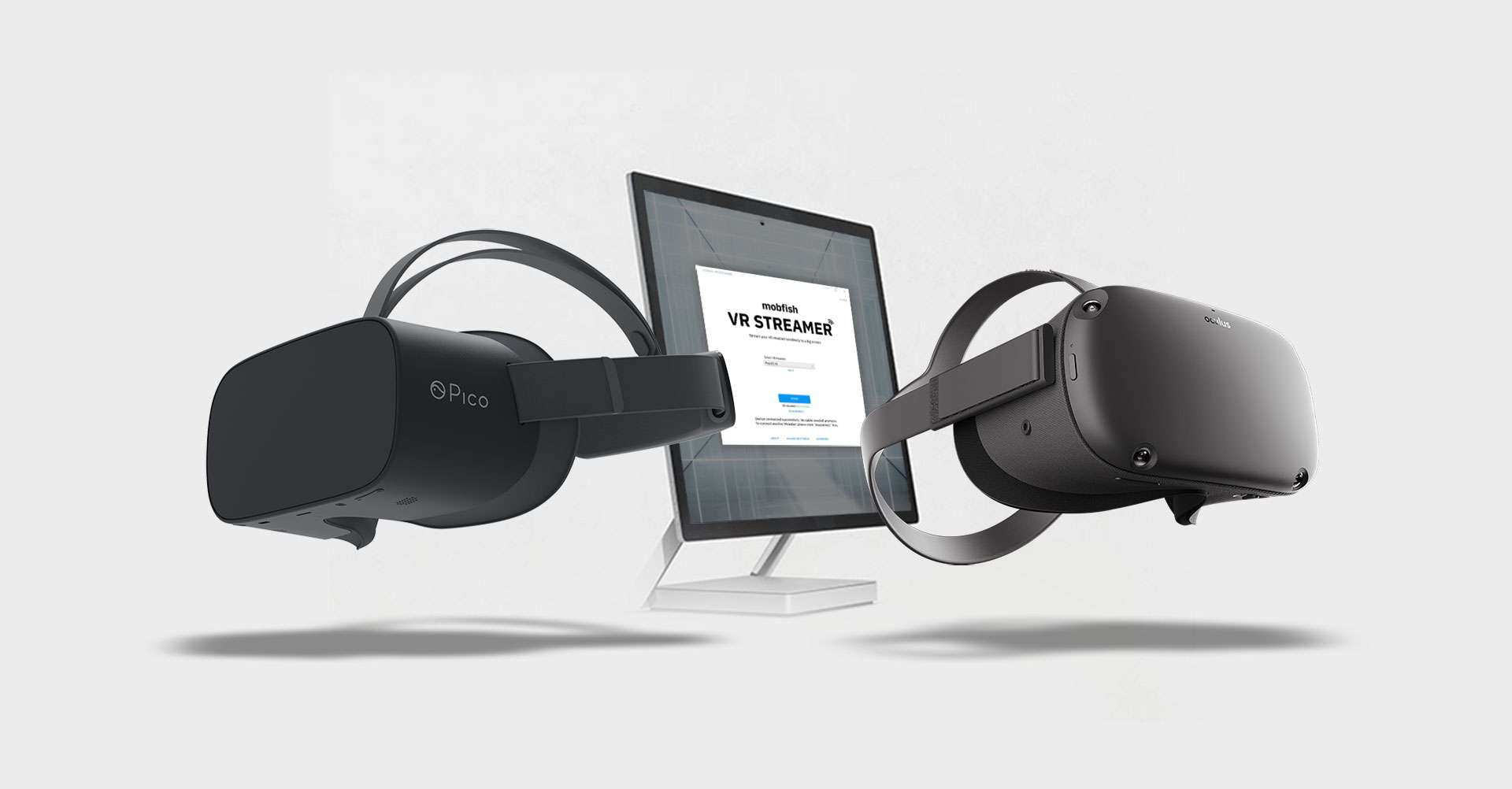The image features a promotional setup for two VR headsets from the brand Pico. Both headsets are black with a matte finish and have adjustable straps designed to secure the device over the eyes, top of the head, and around the back of the neck. The left headset has its straps positioned upwards, showcasing their adjustability, while the right headset is protected by a lens cover. In the center background, a computer monitor prominently displays a white label reading "VR Streamer" against a light gray backdrop. The arrangement appears to simulate the headsets floating, with their shadows subtly visible below, enhancing the display's visual appeal.